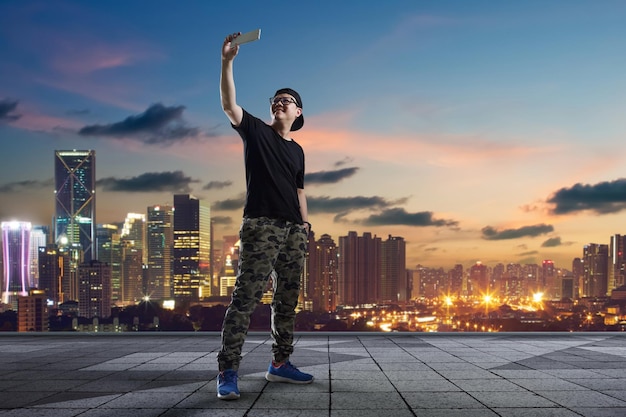A young Asian man is taking a selfie, holding his smartphone high above him, standing on a paved rooftop with square paver tiles. Dressed in casual streetwear—black t-shirt, camouflage skinny jeans, blue sneakers, black horn-rimmed glasses, and a backwards baseball cap—he captures himself in front of a stunning cityscape. The modern city skyline boasts tall skyscrapers with illuminated interiors as night begins to fall. The sky, a tapestry of dark blues and vibrant strips of pink and purple, reflects the last light of dusk with scattered clouds enhancing the scene. The photograph beautifully contrasts the city's bright lights and the fading colors of the sunset, encapsulating the magic hour where day meets night.